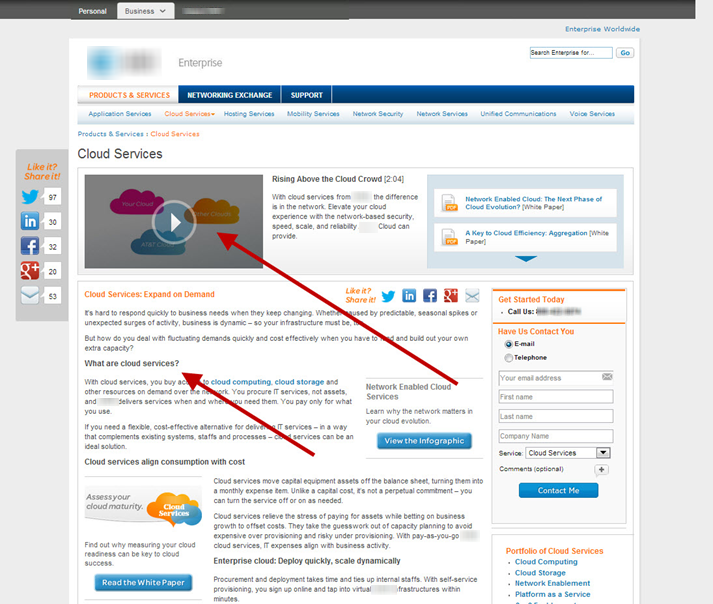Here's a cleaned-up and detailed caption for the image described:

---

The screenshot displays a webpage dedicated to cloud services, set against a minimalist white background. The page features a dark blue text header in the upper left corner stating "Cloud Services." Adjacent to this heading is a YouTube-style video play button within a rectangle, showing a preview with three multicolored cloud diagrams in red, blue, and yellow. The video caption reads, "Rising above the cloud crowd, 204. With cloud services from [redacted], the difference is in the network. Elevate your cloud experience with a network-based security, speed, scale, and reliability that [redacted] cloud can provide."

The page includes several blue clickable buttons for additional features, and two large red arrows are present: one guides the viewer from a "View Infographic" button toward the video, and another directs attention from the lower middle of the page to the main heading.

To the upper right, a pale blue rectangular section offers two downloadable PDF white papers titled, "Network-enabled Cloud: The Next Phase of Cloud Evolution?" and "A Key to Cloud Efficiency Aggregation." These resources provide in-depth information about cloud technology advancements.

In the middle right section of the page, there is a "Get Started Today" section highlighted in an orangish-red color. This area encourages users to sign up by providing their email address, name, company name, and selecting from a dropdown menu listing cloud services. Contact options include phone and email, although the phone number is redacted.

While the page is text-heavy, with detailed descriptions scattered throughout, it maintains a neat layout, supporting users in exploring the extensive services offered.

---